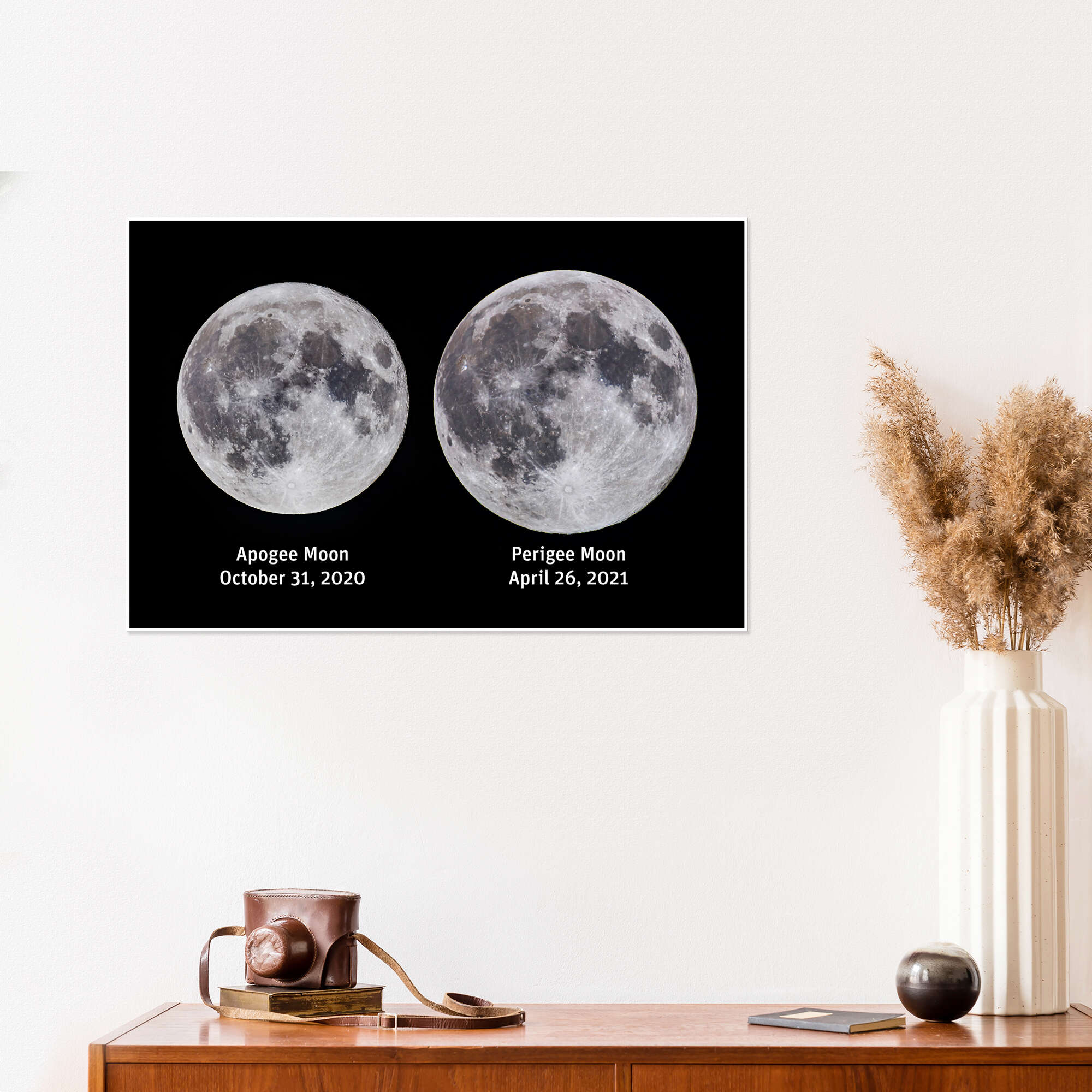The image depicts a wooden shelf against a white wall. On the right side of the shelf, there is a tall white vase containing dried, wheat-like plants that are brownish in color. Next to the vase, there is a small metal ball and a small black notebook. To the left of these items sits a book with what appears to be a vintage camera on top, enclosed in a leather carrying case. The background wall features a black rectangular frame with a white border, displaying two black-and-white moon images. The left image, labeled "Apogee Moon, October 31, 2020," shows a smaller moon, while the right image, labeled "Perigee Moon, April 26, 2021," depicts a slightly larger moon.